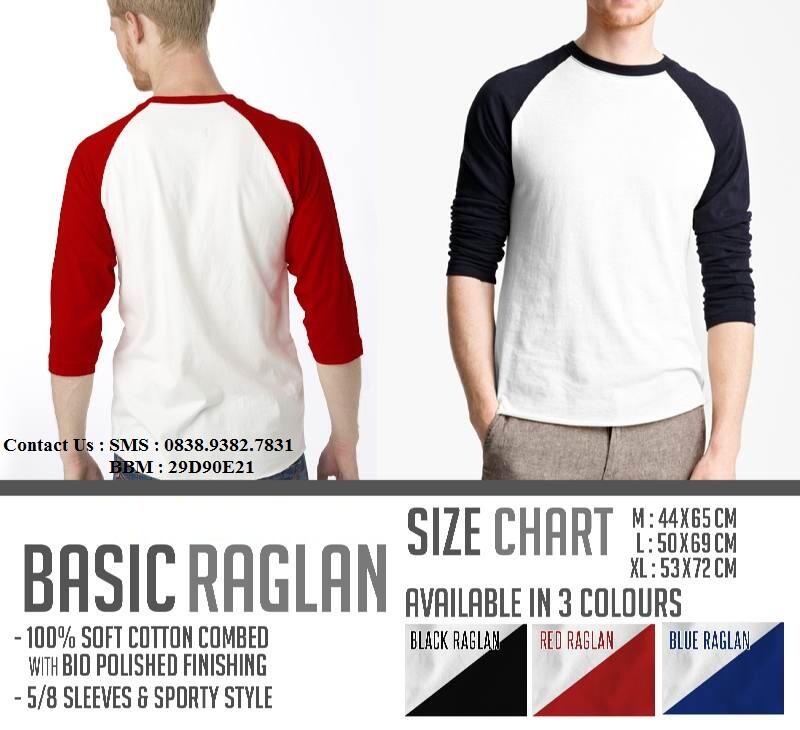The advertisement features a landscape-oriented image promoting a "Basic Raglan" shirt, prominently showcasing two versions of the shirt in different colors. The model, a man with dirty blonde hair, appears twice: on the left, facing away from the camera to display the back of a red-sleeved raglan shirt with a white torso and elbow-length sleeves, and on the right, facing the camera with his hand in his pocket, wearing a black-sleeved version of the same style.

The shirt is detailed to be made of 100% soft cotton with a bio-polished finish. It features five-eighths sleeves and a sporty style. Available in three colors—black, red, and blue raglan—the ad includes a size chart for medium (44 by 65 cm), large (50 by 69 cm), and extra-large (53 by 72 cm) sizes.

Text overlays provide contact information with "CONTACT US: SMS: 0838-9382-7831" and "BBM: 29D90E21." The lower third of the image elaborates on the product features and available options, maintaining a clean, sans serif font for clarity.